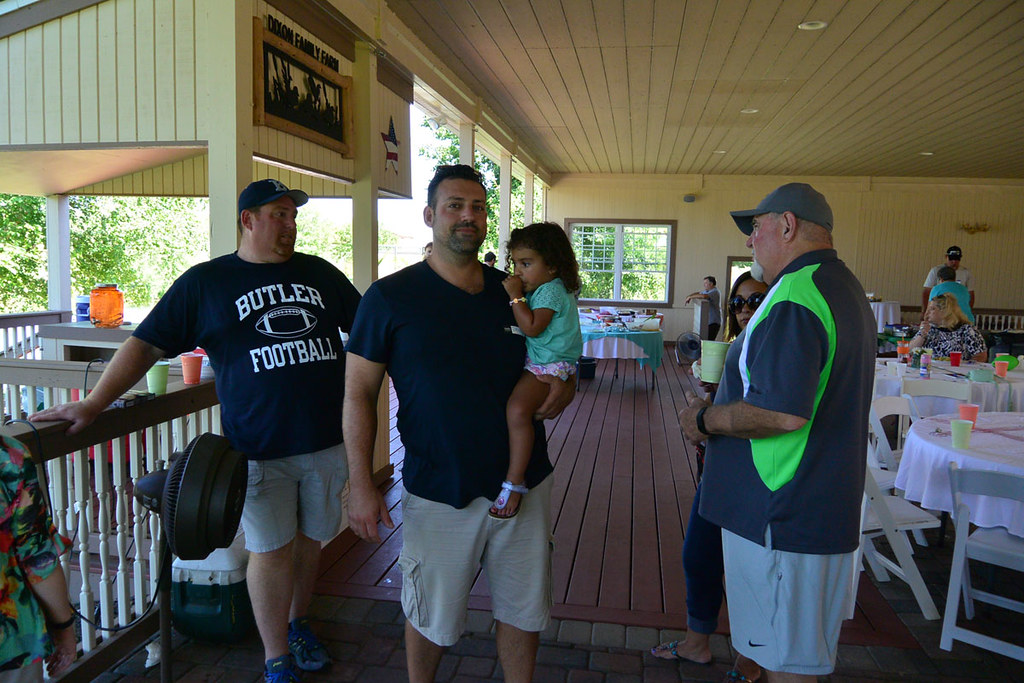The photograph features a covered, open-air restaurant area with a large porch and a wooden floor and ceiling. Dominating the scene are three men standing in the foreground. The man on the left is heavyset, wearing a dark blue T-shirt and a matching baseball cap, both featuring “Butler Football” in white letters, and he stands behind a black floor fan. Central to the image is a man with short brown hair, a trimmed beard, and a blue T-shirt with gray shorts. He is holding a little girl, approximately two years old, with shoulder-length dark brown curly hair and her left hand up to her mouth. To the right, another man is looking towards the first man, dressed in a blue and green polo shirt, white Nike shorts, and a blue baseball cap, holding a drink in his right hand. Partially visible to his right is a woman wearing sunglasses. The background reveals tables set with white tablecloths and colorful cups, suggesting a gathering or event, with a few people seated. The space is open on the left side, offering a view of trees and brown stair railings with white vertical poles. The atmosphere is bright and airy, with the yellow ceiling and the visible window on the far wall enhancing the inviting ambiance.